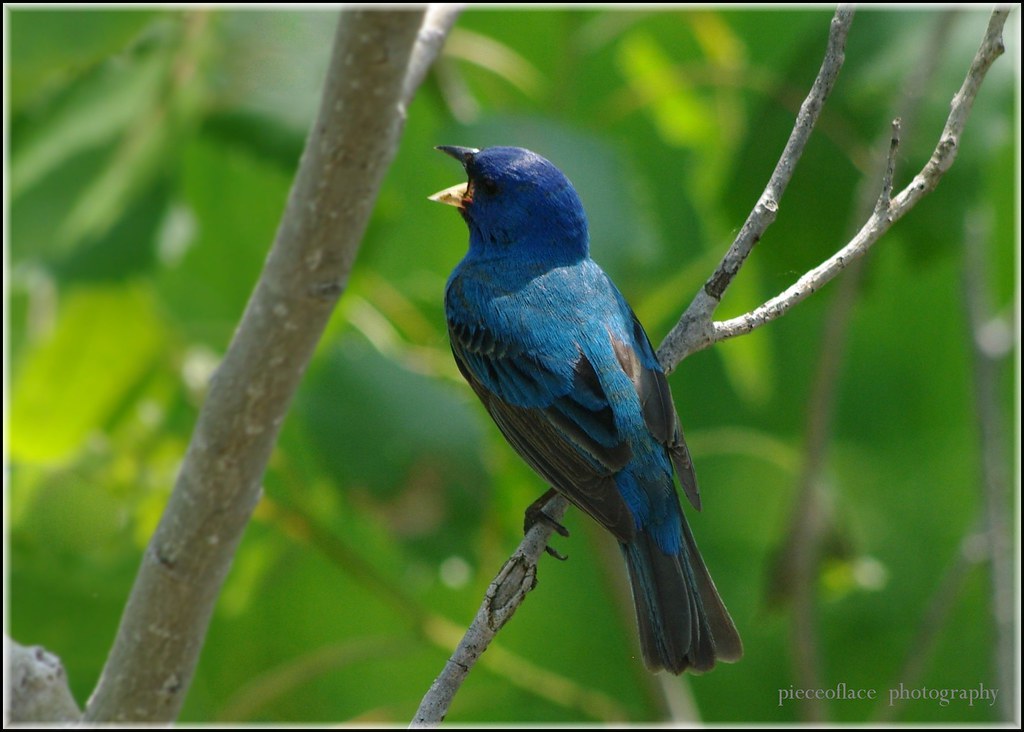This photograph captures a small blue bird, likely a blue jay, perched on a thin, tan-colored branch amidst a blurred backdrop of large green leaves. The bird’s head is a dark, vibrant blue, gradually lightening as the color transitions to the back and wings. It features a mix of blue and dark gray feathers, with black predominant on the tail feathers. The bird’s beak is short and pointy, black on the top and yellowish on the open bottom, possibly due to lighting effects. Its tiny black feet grasp the thin branch securely. The bird's body faces the upper left-hand corner of the image, while its head is slightly turned to the left with its beak open, possibly mid-song. In the bottom right-hand corner, there's text that reads "Pickle Flacko Photography."